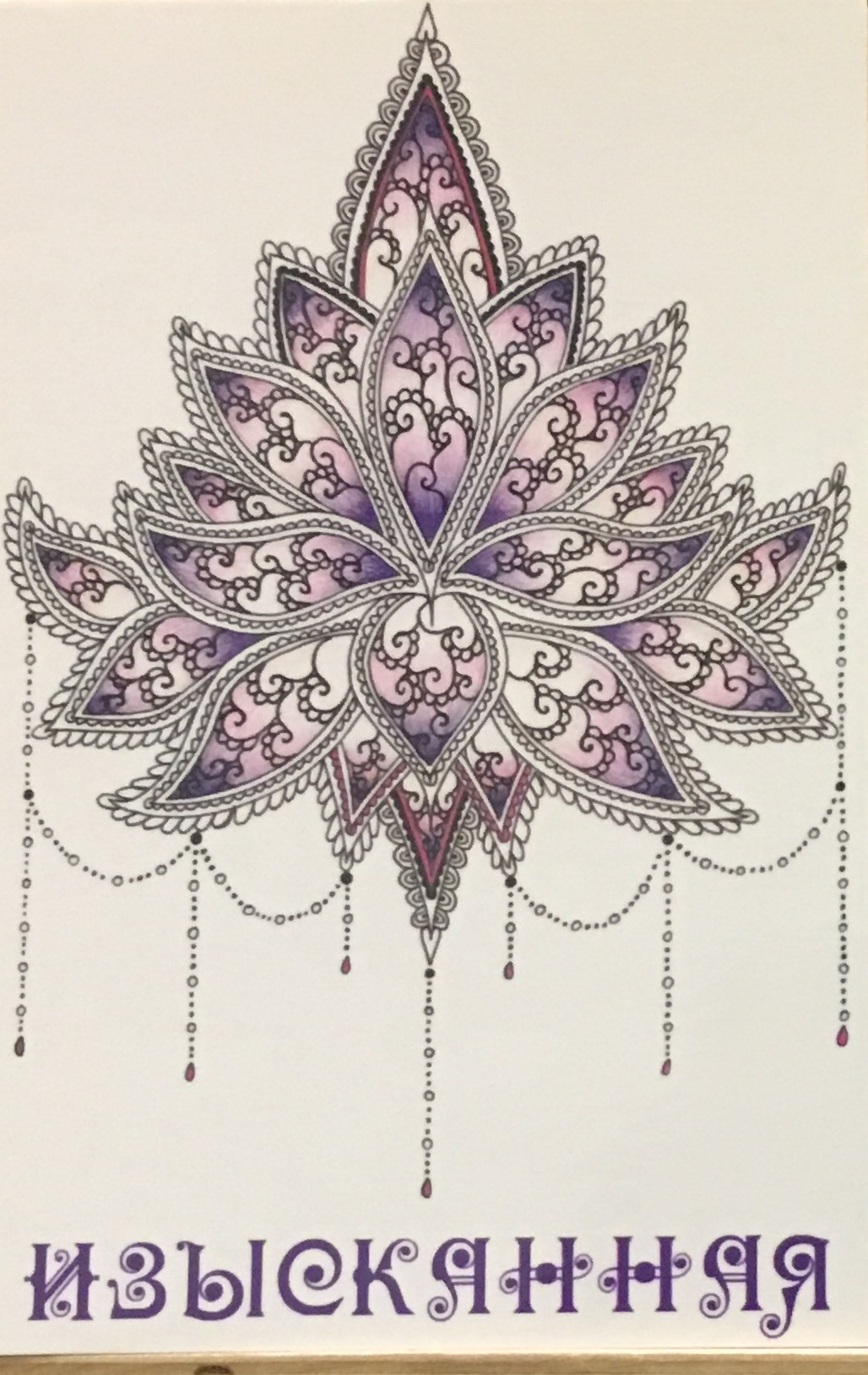The image appears to be an artistic representation of a flower, though not one found in nature. The design features multiple petals, each intricately crafted with unique curves resembling half circles or half ovals. The petals exhibit a gradient color scheme, transitioning from dark purple to medium pink to light pink, ultimately fading into white. The internal curves within each petal further enhance their elaborate design.

Beneath the flower, there is a caption written that bears a resemblance to a Sanskrit word. Additionally, small decorative chains or links hang down from some of the petals, creating an interconnected visual effect. These chains add to the overall elegance of the piece.

The flower appears to be positioned on a surface of varnished wood, possibly indicating that it is displayed on an easel or another wooden platform, providing a refined and polished base for the artwork.